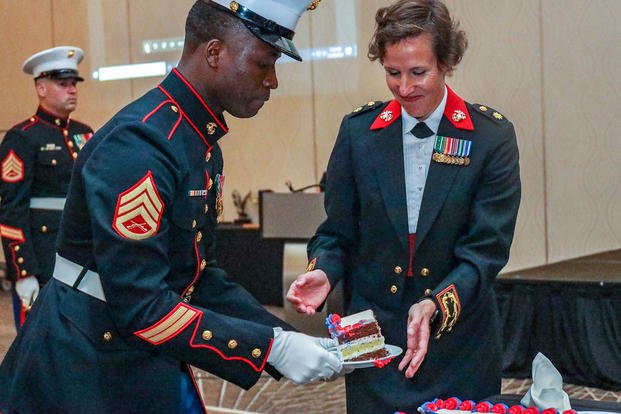The image depicts a formal Marine celebration, clearly a ceremonial event given the presence of senior Marine NCOs in full dress blue uniforms adorned with numerous medals and emblems, complete with white gloves. The room features several tables draped in black tablecloths, adding to the formal ambiance. Central to the scene is a beautifully decorated cake, with white frosting and red, white, and blue trim, suggesting a patriotic theme. One senior Marine NCO is in the act of serving the cake, donning a white hat and exhibiting red piping and a red belt as part of his uniform. He serves a piece to a female Marine officer, who also wears a dress blue uniform but without a hat or gloves. Her uniform indicates her officer status through distinct collar medallions. The details and coordination of the uniforms and decorations imply a significant and respectful observance, possibly honoring the woman's service or marking a notable occasion for the Marines.